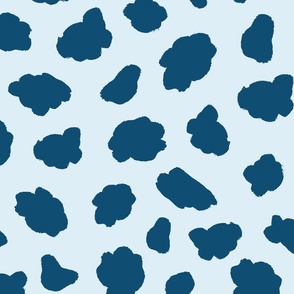This abstract illustration features a square canvas with a light blue background, adorned with approximately 20 dark blue, cloud-like shapes evenly distributed throughout the image. The cloud shapes are all distinct yet share an abstract, fluffy appearance, reminiscent of doodles or stylized clouds. The color palette is simple and consistent, with the dark blue shapes adding a striking contrast to the lighter blue backdrop. The overall design creates a graphic pattern with a playful, yet orderly feel, characterized by its abstract simplicity and repetitiveness.